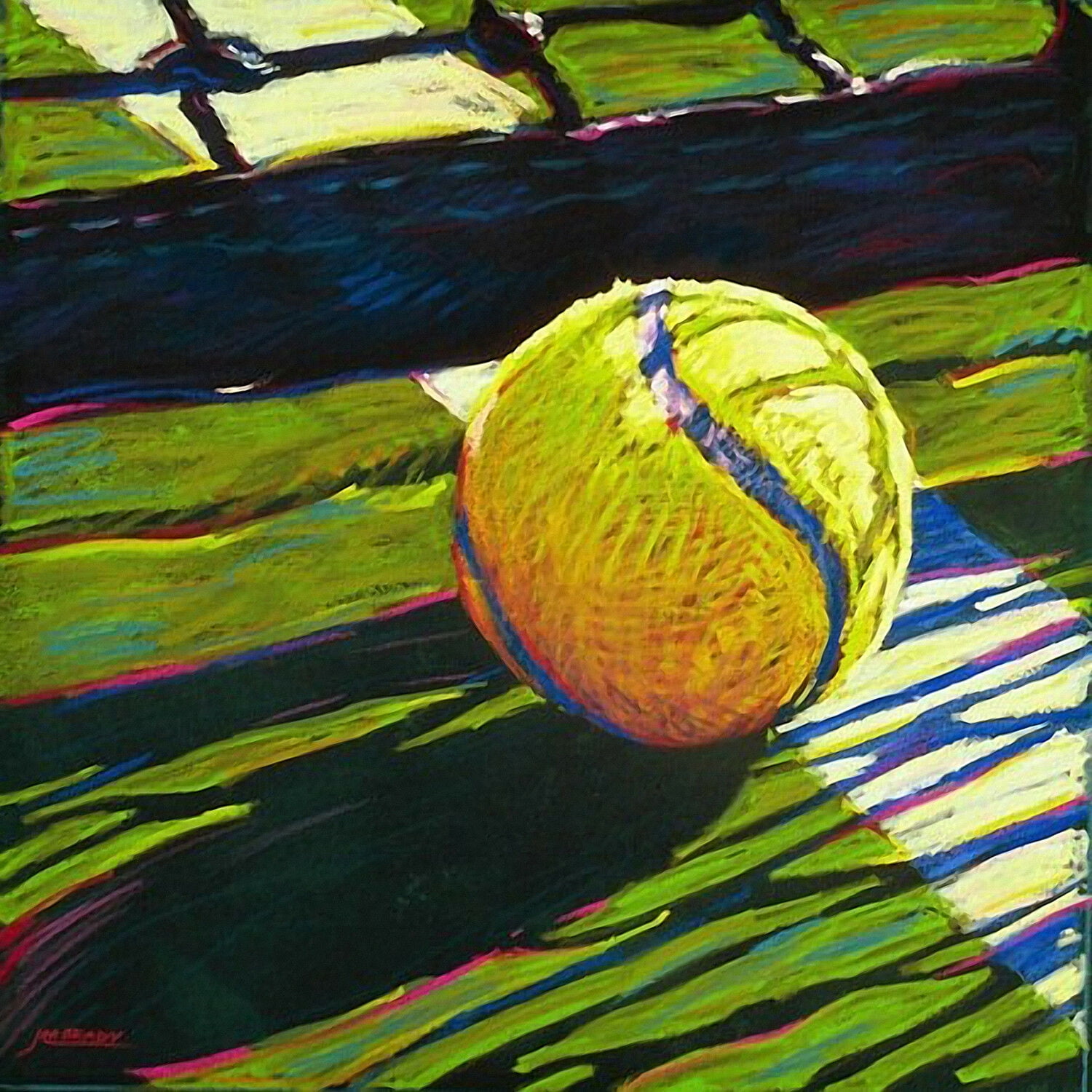This painting prominently features a tennis ball characterized by a bright yellow hue with a contrasting blue line, positioned dynamically on a tennis court. The court itself is green with intricate shadow play, including deep purples, blues, reds, and oranges, rendering a sense of depth and movement. The tennis ball is depicted with meticulous detail, showcasing its textured threads and sitting on a surface striped in yellow and blue, with the bottom part cast in shadow and the top illuminated. The image captures a moment where the ball appears ready to bounce just inside the inbounds line. Above the ball, the bottom part of a tennis net is faintly visible, partially obscured by shadows that suggest the presence of people standing nearby. The painting employs a line-heavy, dynamic style that imbues the still image with an impression of motion and energy.